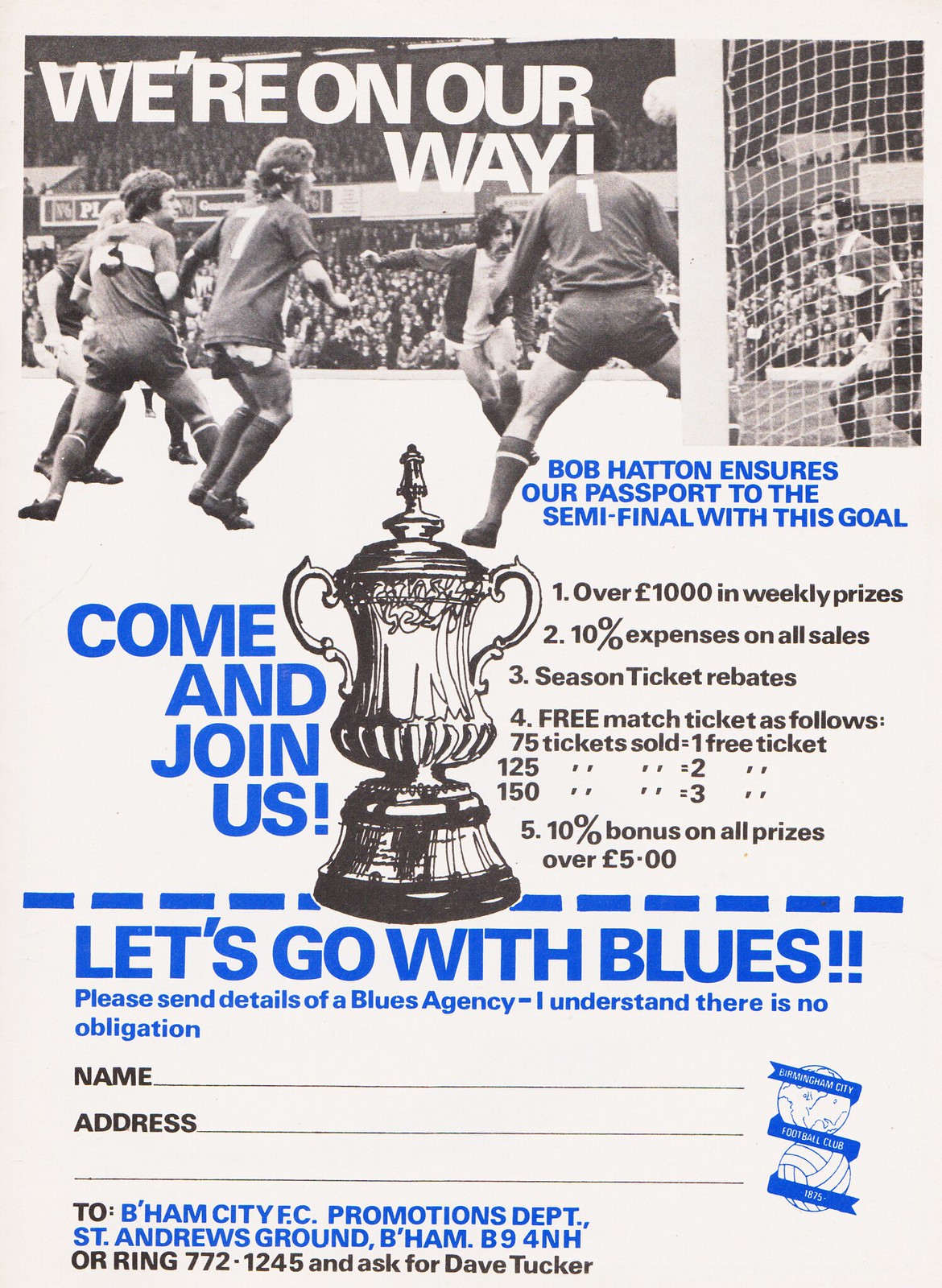The image is a vintage advertisement flyer, likely from the 1980s or 1990s, promoting a football (soccer) event. It is rectangular in shape, featuring a black and white photograph across the top, capturing a live-action moment of a soccer match. In the image, a player, Bob Hatton, is about to score a goal amidst a crowd of defenders, with the stadium stands packed with spectators in the background. 

The top of the flyer prominently displays the text "We're on our way" in white, followed by "Bob Hatton ensures our passport to the semifinal with this goal" in blue. Below this, another line in blue invites people with "Come and join us." Accompanying the text is an illustration of a trophy, symbolizing the competitive spirit of the event.

Further down, the flyer lists enticing offers and incentives:
- Over £1,000 in weekly prizes
- 10% expenses on all sales
- Season ticket rebates
- Free match tickets for selling a certain number of tickets (e.g., 75 tickets sold equals one free ticket, 125 equals two, 150 equals three)
- A 10% bonus on all prizes over £5

At the bottom of the flyer, there's a cutout section encouraging fans to join with a call to action: "Let's go with Blues." This section includes a form where individuals can request details about a Blues agency, ensuring there is no obligation, with spaces provided for their name and address, and the address to send the ballot to.